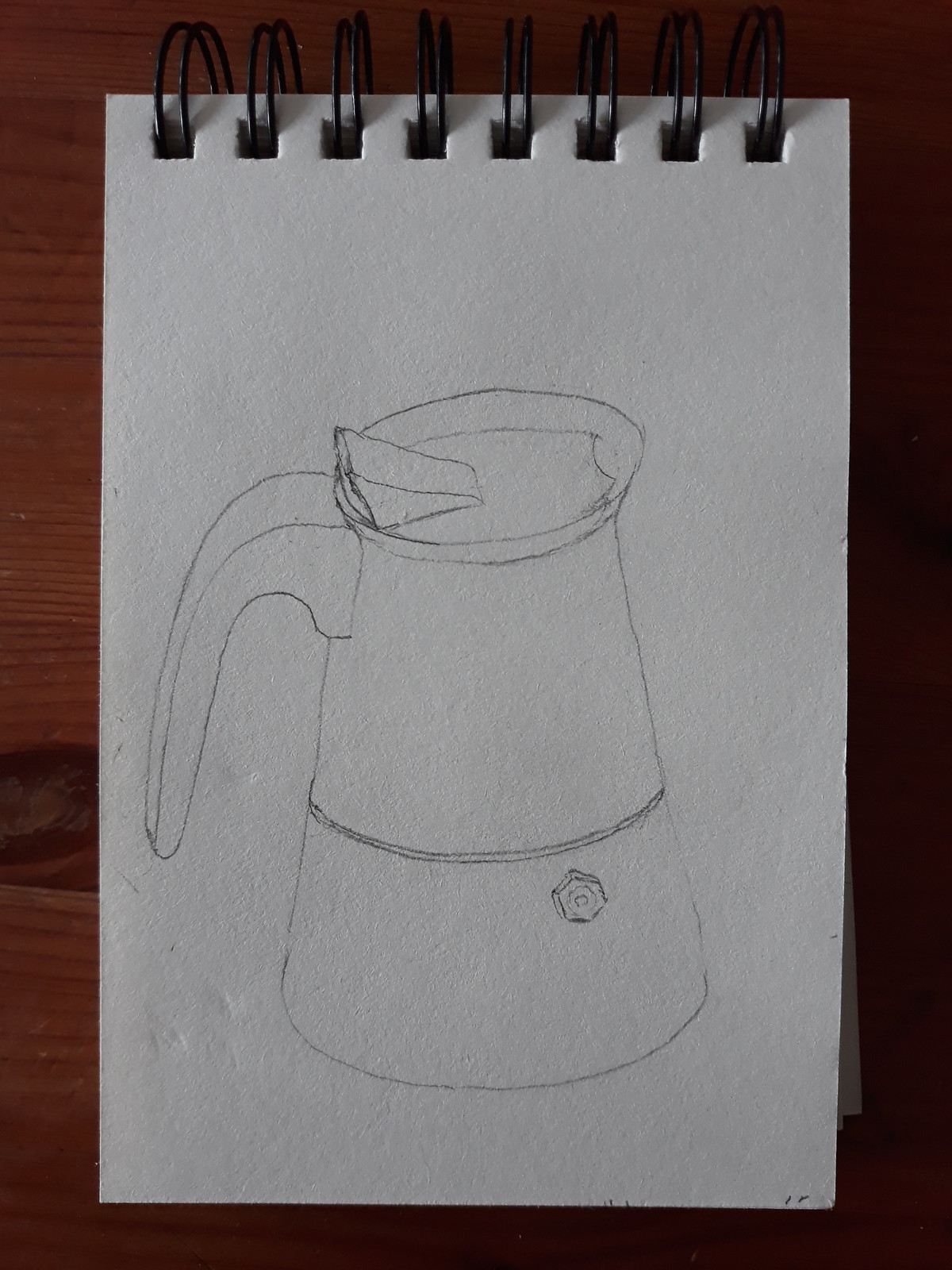The image features a simple black ink line drawing of an old-style coffee pot or electric kettle created on plain white paper in a small, hand-held sketchpad with a ring binder at the top. The sketchpad rests on a cherry oak wooden table. The pot is cylindrical with a wider base than its top, and it has a long handle attached at the top that resembles a tail. There is a distinct pouring spout on the lid, and a line around the middle of the pot. The drawing includes minimal detailing, no signatures, and some faint indentations or dust marks. The overall photograph is somewhat dark.